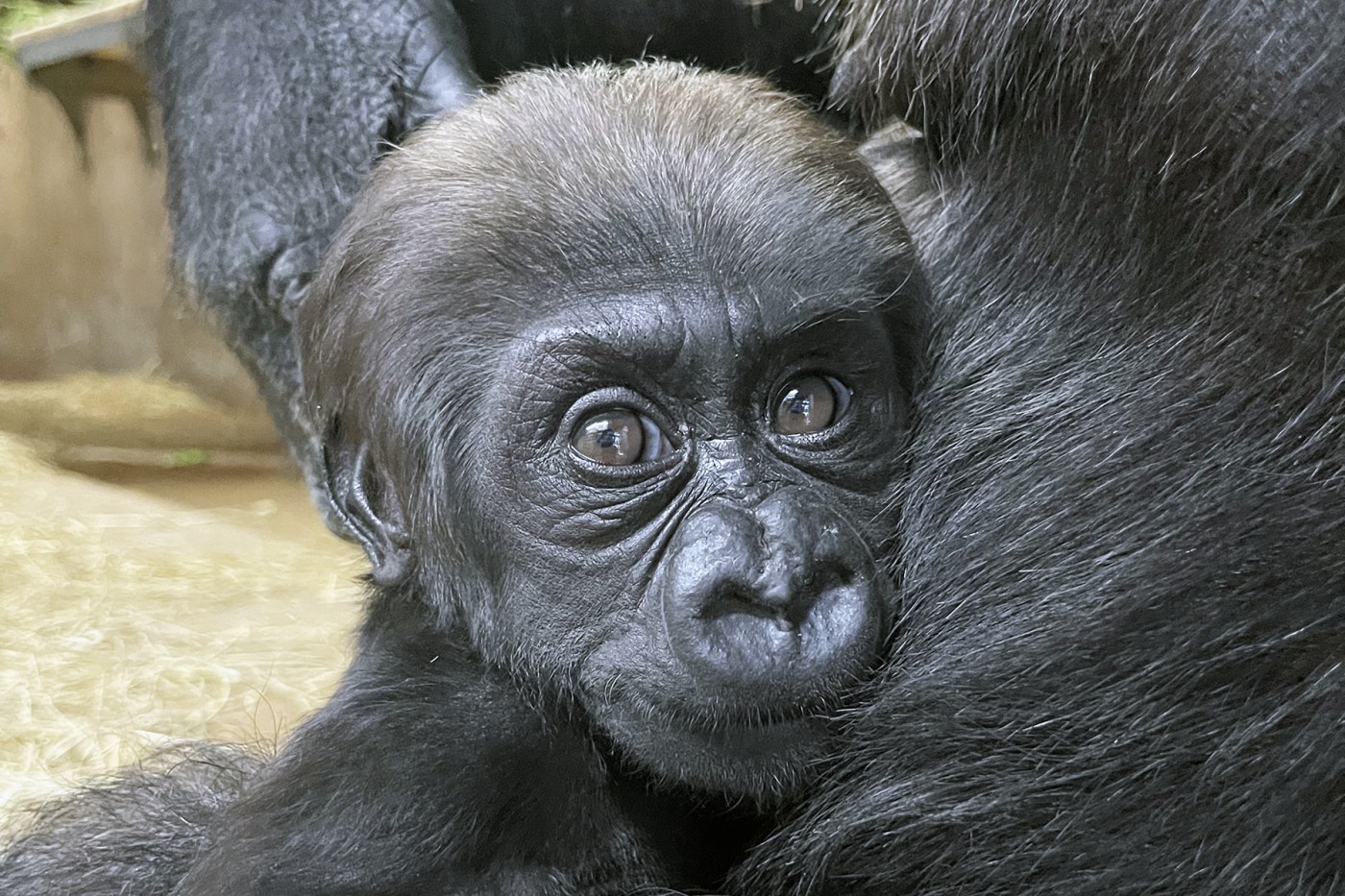A high-quality photograph captures a tender moment between a baby gorilla and its presumably mother in what appears to be a barn setting. The focus is primarily on the baby gorilla, whose large, expressive brown eyes and broad nose are clearly visible. Its dark fur covers most of its face, and the small, stubby ears frame its head, with the right ear more prominent while the left ear is pressed against the mother's chest. The baby’s fur, which ranges from a deep black on the body to a golden brown on top of the head, contrasts slightly with the mother's darker fur. The mother's presence is mostly suggested by the dark hair and her comforting embrace. You can see her hand gently cradling the baby’s head and part of her right arm from shoulder to elbow. The surrounding environment includes a bed of yellow hay to the left and a slightly out-of-focus shelf in the background, offering a cozy and intimate glimpse into their habitat. The baby gorilla's face, gazing wide-eyed at the camera, is the central focus, radiating a sense of innocence and security in its mother's arms.